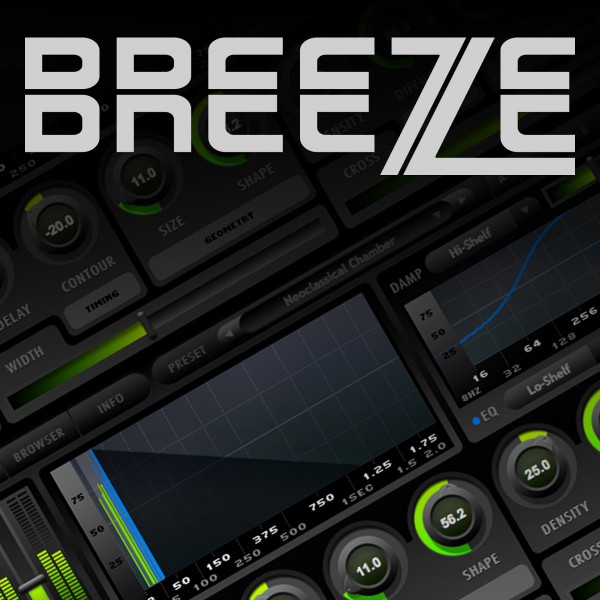The advertisement for Breeze features a digital dashboard of what appears to be a music or audio editing software, displayed in a detailed graphic image. The background is predominantly gray and black, with numerous dials and charts showcasing aspects like shape, density, contour, delay, and size. The interface also displays numerical values on the dials, such as 56.2 for density and 25.0 for another setting. Lime green and blue accents indicate different settings and levels, with lime green specifically showing the extent to which a dial is turned. Blue lines map out the contours in the line charts. Superimposed on the interface in a striking white font, the word "BREEZE" is prominently displayed. The font is unique, with each letter bisected horizontally, making the Z resemble a seven and an L. The overall design exudes a modern, tech-savvy vibe, likely appealing to enthusiasts and professionals in audio editing or mixing.